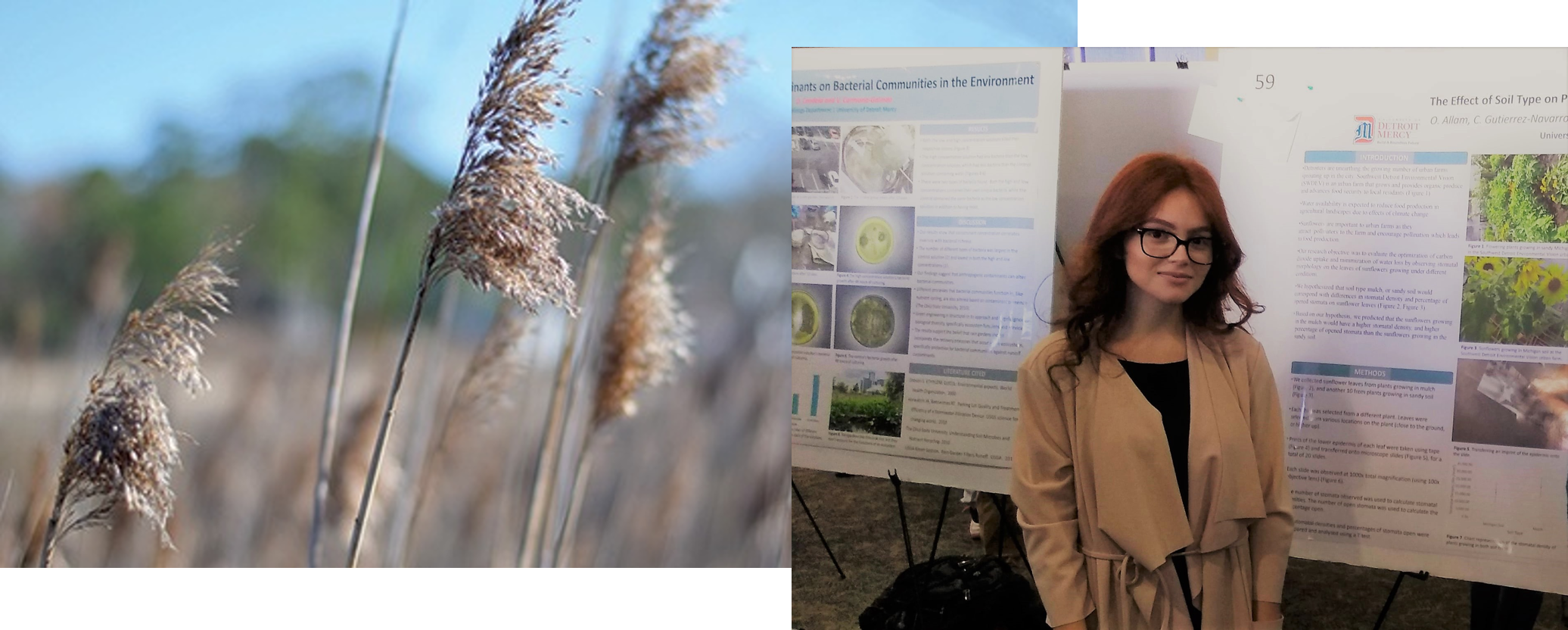This composite image features two overlapping photographs. The larger, horizontally aligned rectangular photo on the left captures a close-up view of tall blades of grass, characterized by their brown, feathery tips. In the blurred background, green trees and a hint of blue sky can be seen, suggesting a natural, outdoor setting. The overlapping square-shaped photo on the right portrays a young Caucasian woman with long, wavy, reddish-brown hair, smiling at the camera. She is wearing black, round glasses, a black shirt, and a tan-colored coat. She stands in front of two large, white poster boards mounted on black stands, each displaying various images, text, and charts related to environmental topics. The legible part of one poster reads, "The effect of soil type on...," while the other mentions "bacterial communities in the environment," indicating that she is likely presenting scientific research on these subjects.